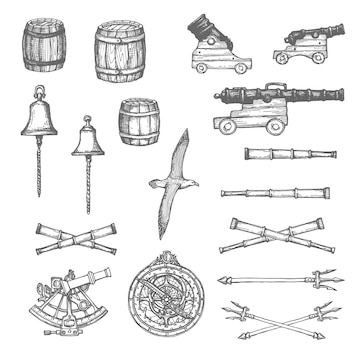This black-and-white diagram comprises several detailed sketches. In the top left corner, there are three barrels followed by two bells hanging below. Just beneath the bells, a bird, possibly a seagull, is depicted with its wings fully stretched. Directly below the bird is a compass. On the right side of the image, there are various wooden vehicles resembling carts equipped with cannons. Additionally, there are a few telescopes and swords; some swords are crossed, forming an X. In the bottom left corner, we see a vintage protractor and two bamboo sticks arranged in an X-shape. There are also miscellaneous elements like pitchforks and more telescopes scattered throughout the composition. All these detailed items are intricately sketched, likely with pencil, contributing to the diagram’s rich and historical aesthetic.